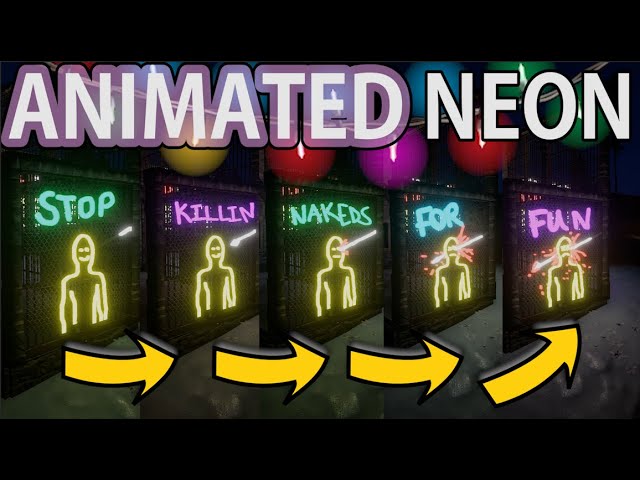The image displays a horizontal sign with a black background. At the top, in thick, all-capital letters, it reads "ANIMATED" in white font with a translucent purple border, followed by the word "NEON" in white. Below the text, there are five sections framed by yellow arrows pointing to the right, creating a connected sequence. Each section features a human figure outlined in bright lights. The first section shows the word "STOP" in green above a smiling figure. In the second section, labeled "KILLING" in pink, an arrow approaches the figure. The third section says "NAKEDS" in green, where the arrow makes contact with red lines indicating injury. The fourth section with "FOUR" in blue displays the arrow piercing through the figure, who now has a distressed expression. The final section, labeled "FUN" in purple, shows the arrow completely through the figure, who has x's for eyes and a fully frowning face. Additional details include various colored balloons beneath the text "ANIMATED NEON," contributing to the chaotic yet engaging visual narrative.